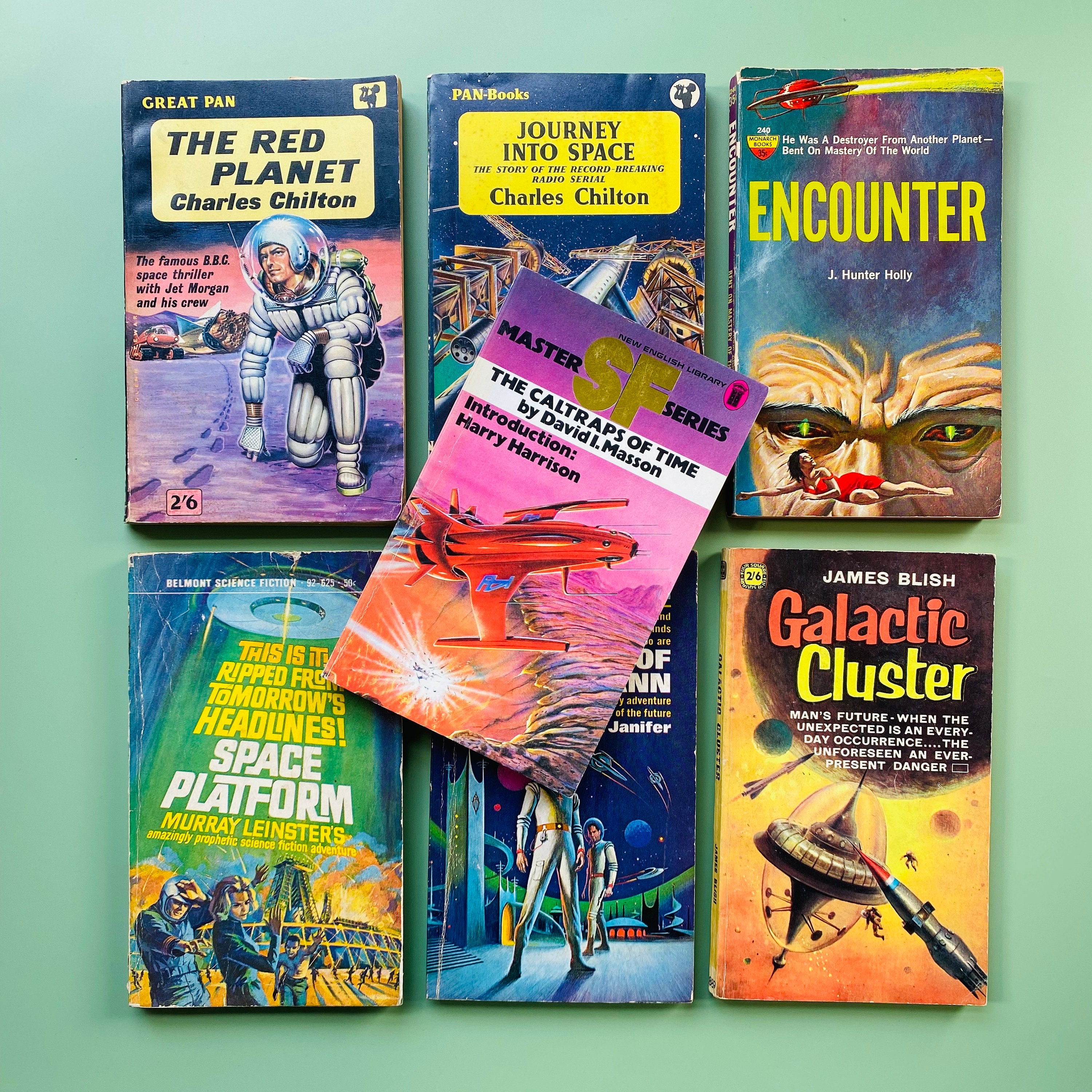The photograph showcases a collection of seven classic science fiction paperback books arranged against a light blue background. They appear to be older publications, likely from around the early 1960s. The books are organized in two rows of three, with an additional book lying on top, slightly covering some of the titles.

In the top row, from left to right:
1. "The Red Planet" by Charles Chilton, featuring an astronaut on its cover.
2. "Journey into Space" by Charles Chilton, depicting a satellite.
3. "Encounter" by J. Hunter Hawley, illustrated with a man with glowing eyes and a woman in a red dress.

In the bottom row, from left to right:
4. "Space Platform" by Murray Leinster, with the tagline "This Is It, Ripped From Tomorrow's Headline," showing an alien spaceship and frightened people.
5. An unidentified title, partially obscured by the book on top.
6. "Galactic Cluster" by James Blish, featuring spaceships and rockets and emphasizing mankind's future dangers.

On top of these six lies:
7. "The Caltrops of Time" by David I. Masson, identified as part of the Master SF Series and having an introduction by Harry Harrison. The cover is predominantly pink and suggests a canyon setting.

Common elements across the covers include images of astronauts, spacecraft, and futuristic scenes, reinforcing their shared sci-fi genre.